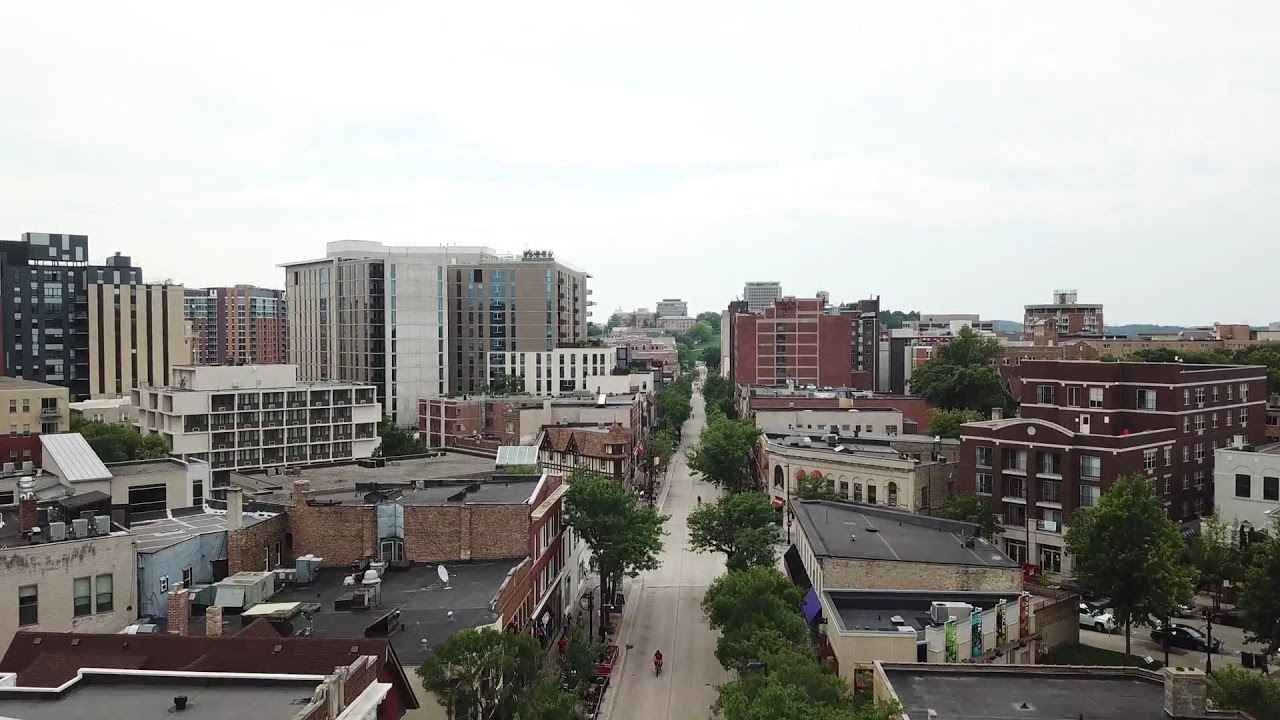This detailed full-color aerial photograph captures a mid-sized foreign city on a cloudy day. The focal point is a light gray concrete street running directly through the center of the image, devoid of traffic but featuring two bicyclists—one pedaling towards the camera and another further away in the opposite lane. The street, possibly four lanes wide with two lanes in each direction, is flanked by green-leafed trees lining both sides. 

To the right and left of the street are densely packed buildings, varying from three-story structures near the forefront to larger, more considerable buildings reaching approximately eight to twelve stories. These buildings are predominantly residential, constructed mainly of brick, with flat rooftops dotted with equipment such as satellite dishes. Among these buildings, smaller municipal structures resembling city council halls are also present. Farther into the distance, a taller building, potentially a hotel, punctuates the skyline, adding to the mixture of architectural heights and styles visible in this urban landscape.